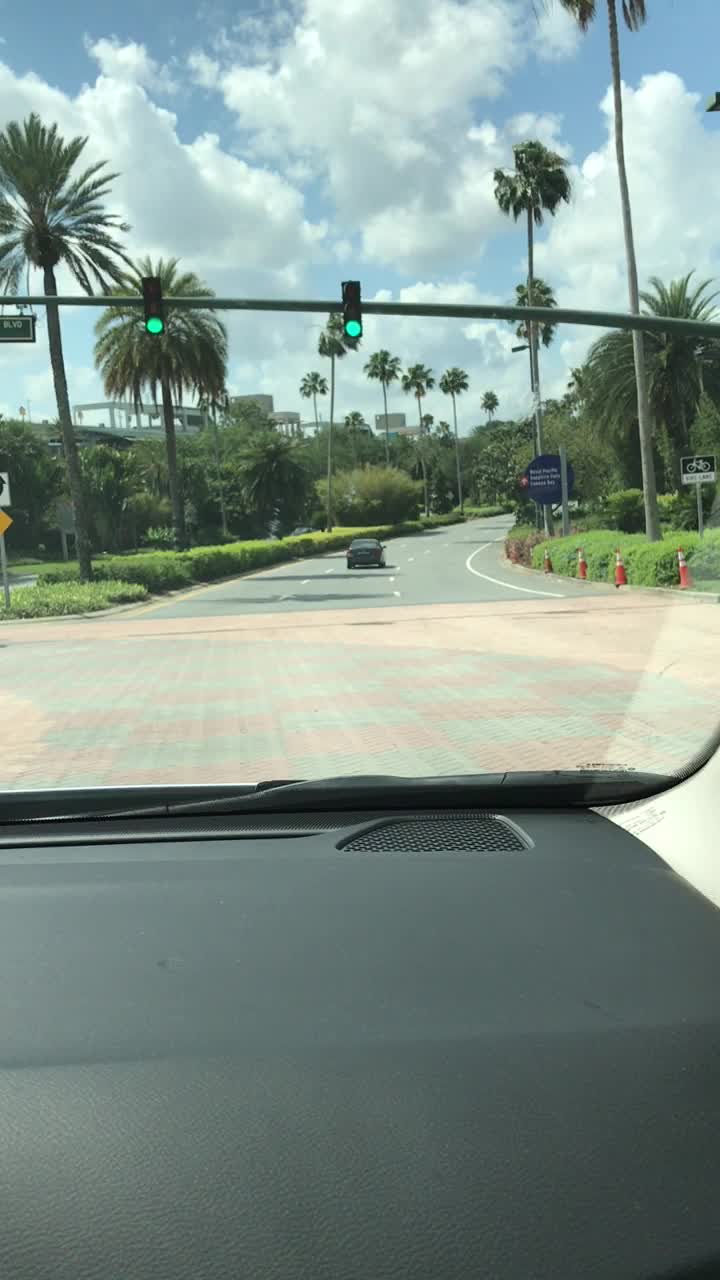In this vertically-oriented photograph, we are presented with a stunning tropical vista as seen from the passenger seat of a moving car. The windshield frames a lush, verdant scene dominated by an array of majestic palm trees lining the road. On the right side, both king and queen palm trees tower over vibrant, green foliage that carpets the ground. In the distance, partially obscured by the trees, an architectural structure - possibly a bridge or a building - is visible, its light gray hue contrasting subtly against the lush environment. Above this picturesque landscape, a brilliant blue sky stretches out, filled with thick, billowy white clouds that add depth and texture to the scene. The car’s solid black dashboard and the right edge of the windshield are visible in the foreground, grounding the viewer in the cozy perspective of a tropical drive.